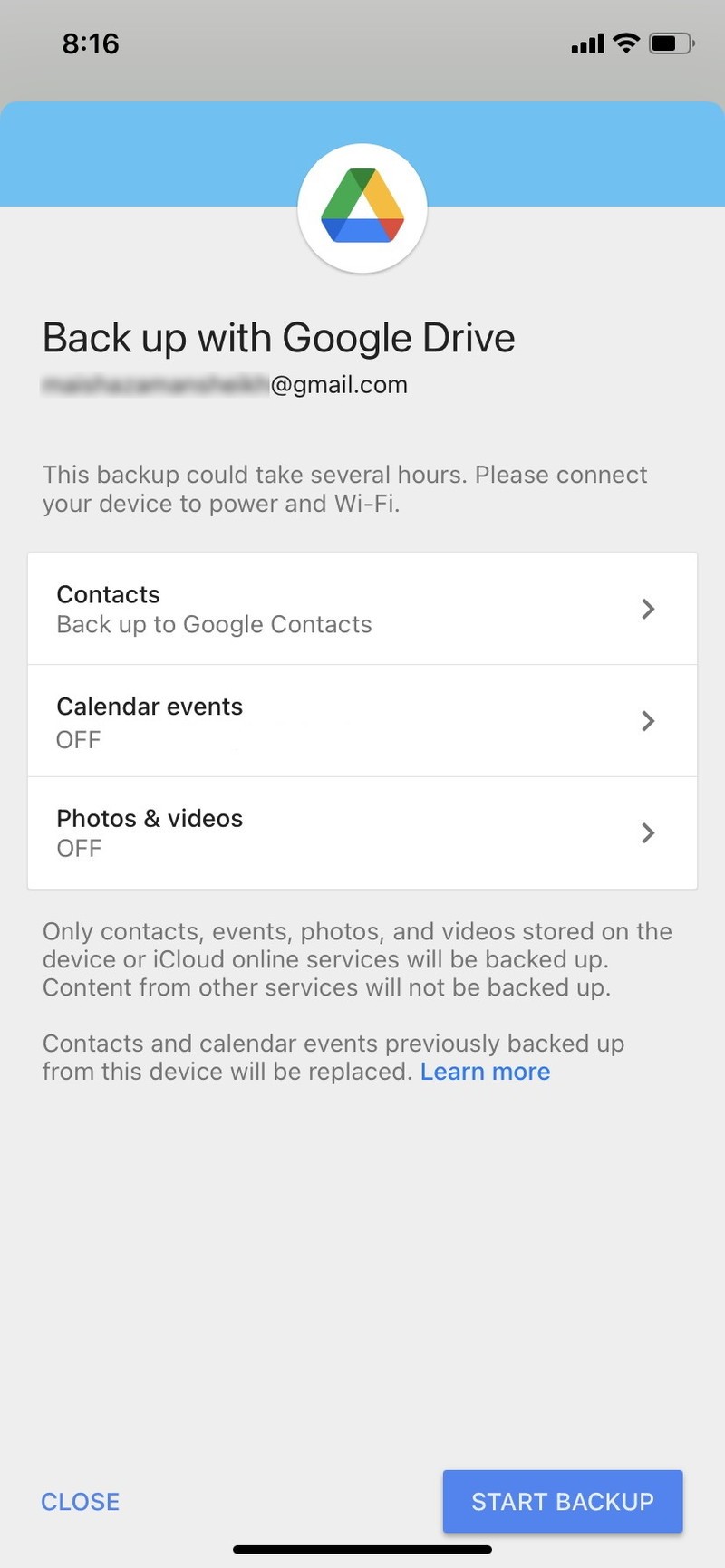A detailed caption for the provided image could be:

"A screenshot of a smartphone's backup settings interface. At the top, the device time reads 8:16, and all signal indicators show full strength — cellular signal bars, Wi-Fi, and battery life. Below this, a blue banner features a circular icon with the familiar Google logo, comprising green, yellow, red, and blue colors arranged in a triangular fashion. Accompanying text indicates 'Backup with Google Drive,' followed by a blurred-out web address ending in '@gmail.com.' A message beneath this advises that the backup process might take several hours and recommends connecting the device to power and Wi-Fi. The interface is divided into sections showing backup options: 'Contacts' is highlighted in a white box with black text, gray subtext notes 'Backup to Google Contacts,' and an arrow suggests further options. Similarly, 'Google events' is listed with black text indicating it's currently 'Off,' and there is a tab to manage this setting. 'Photos and videos' also appear with black text and a gray 'Off' status. At the bottom of the screen are two blue buttons, 'Close' on the left and 'Start Backup' on the bottom right."